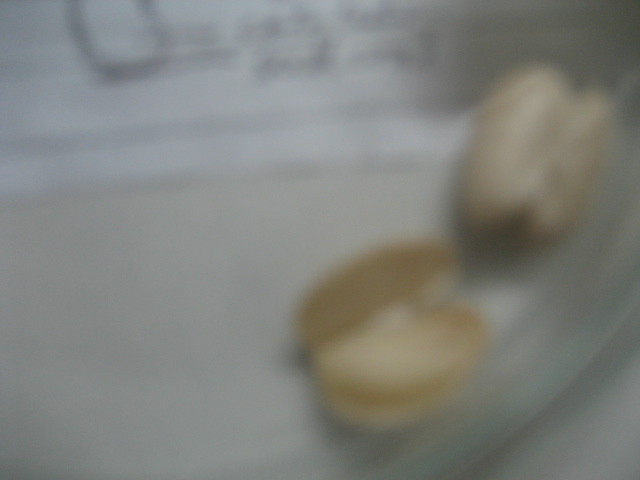The image is a very blurry, rectangular photograph that’s difficult to decipher due to its heavy out-of-focus quality. In the upper portion of the image, there is a white piece of paper which seems to have black text on it, although the writing is too unclear to read. The paper appears to have a black border at the bottom edge and resembles a section where one might sign a contract or letter, giving the impression of an official document, possibly written in cursive.

The background beneath the paper is an off-white, flat surface, likely a table. In the lower right corner, there are two beige, cream-colored objects that resemble clamshell containers or old-fashioned pill bottles from the 1950s. One container is upright and closed, while the other appears to be open with a segment missing, much like the gap in an orange with some sections removed, suggesting potential use for storing items. The objects could also be mistaken for light-colored pistachio nuts with one pried open. Additionally, a flexible, straw-like object is visible nearby, further adding to the mysterious nature of the scene.